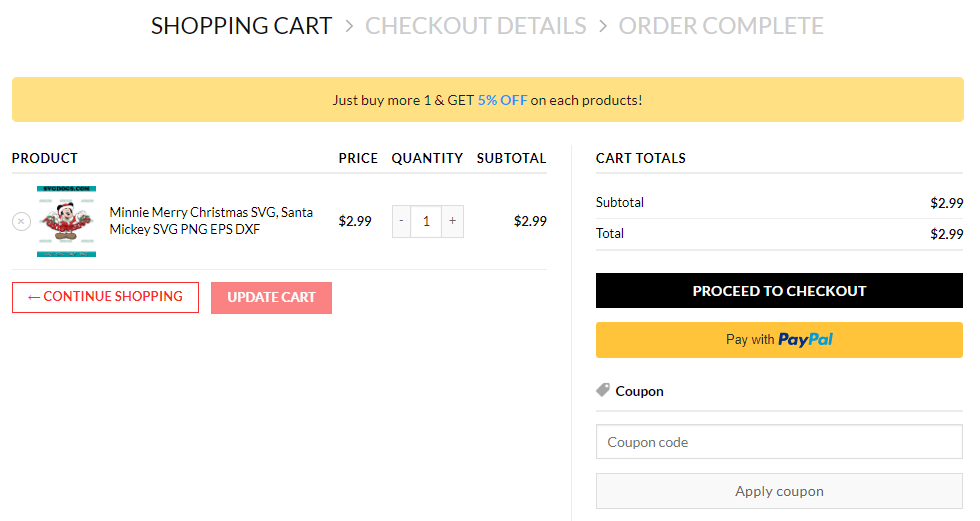The image depicts a shopping cart interface with various detailed elements. At the top, there is a bold headline that reads "Shopping Cart." Below this, in smaller grey letters, there are steps indicating "Checkout Details" and "Order Complete." The header is highlighted in yellow and features a promotional message: "Just buy one more and get 5% off each product."

In the main section, a product listing is displayed, featuring an image of Minnie Mouse dressed in a Santa outfit. The product title reads "Minnie Merry Christmas, SVG, Santa Mickey, SVG, PNG, EPS, DFX," and it is priced at $2.99.

Beneath the product list, there are options to either continue shopping or update the cart. "Continue Shopping" is highlighted in red letters on a white background, while "Update Cart" is displayed in white letters on a red background.

To the right, the cart total section shows both the subtotal and the total as $2.99. Below these figures, there is a black button with white text prompting the user to "Proceed to Checkout." Another option to pay with PayPal is provided, indicated by black text reading "Pay with" followed by the PayPal logo in dark blue and light blue on a yellow background.

At the bottom of the interface, there is a small section with a price tag icon next to the word "Coupon." This section includes a field to enter a coupon code, along with a button to apply it to the order.